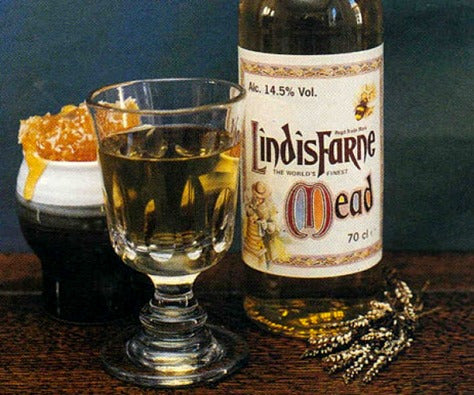The image showcases a bottle of Lindisfarne mead, marked with a white label featuring reddish, yellow, and blue accents, and it states an alcohol content of 14.5%. The bottle, positioned on a brown wooden table with subtle black streaks, stands upright among various objects. In front of the bottle, there is a liquor glass filled mostly with a translucent yellow liquid, presumably the mead. To the left, a small black container with a white top, possibly containing a lumpy, honey-like substance, leaks slightly. Additionally, a cup filled with yellow candy sits beside the container. Scattered near the bottle, there is a metallic object resembling keys, though it's not entirely clear what they are. The scene is set against a blue background, possibly a wall or the interior of a bar, enhancing the contrast and details of the objects on the table.